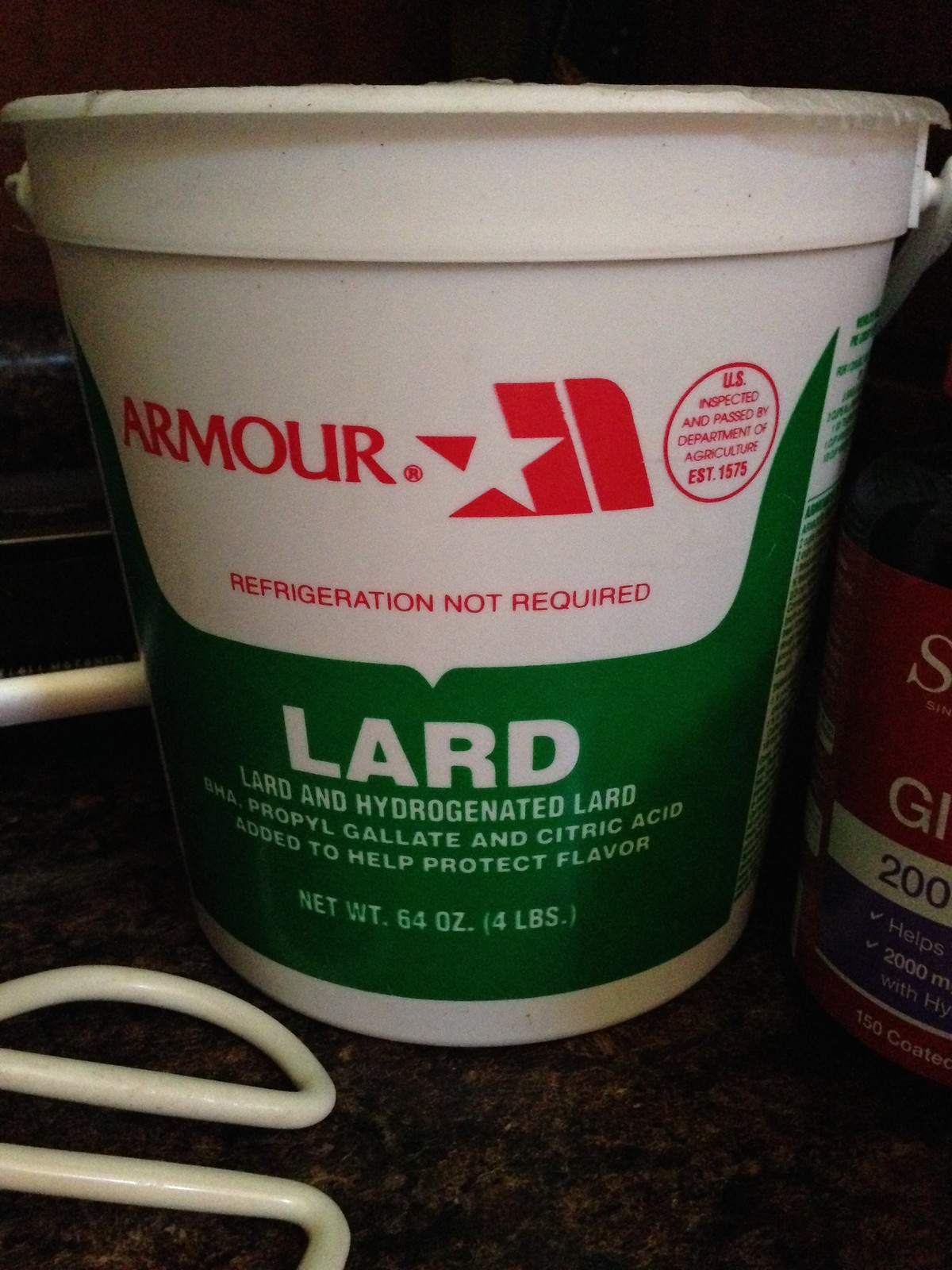The image is a close-up of a white and green plastic tub of lard resting on a brown textured countertop. The container features a prominent red logo that includes the word "Armour" with a star symbol, and below it is an inscription that reads "Refrigeration Not Required." To the right, a red circular seal indicates "U.S. Inspected and Passed by Department of Agriculture Established 1575." The green lower part of the tub prominently displays the word "LARD" in large white letters, followed by smaller text that reads "Lard and Hydrogenated Lard. Propyl Gallate and Citric Acid added to help protect flavor." The container has a net weight of 64 ounces (4 pounds). Adjacent to the tub, on the same countertop, are what appear to be the white handles of a pair of scissors or tongs, and a glimpse of another item to the right which includes part of a bottle showing the number 200 and partial letters GI and S.